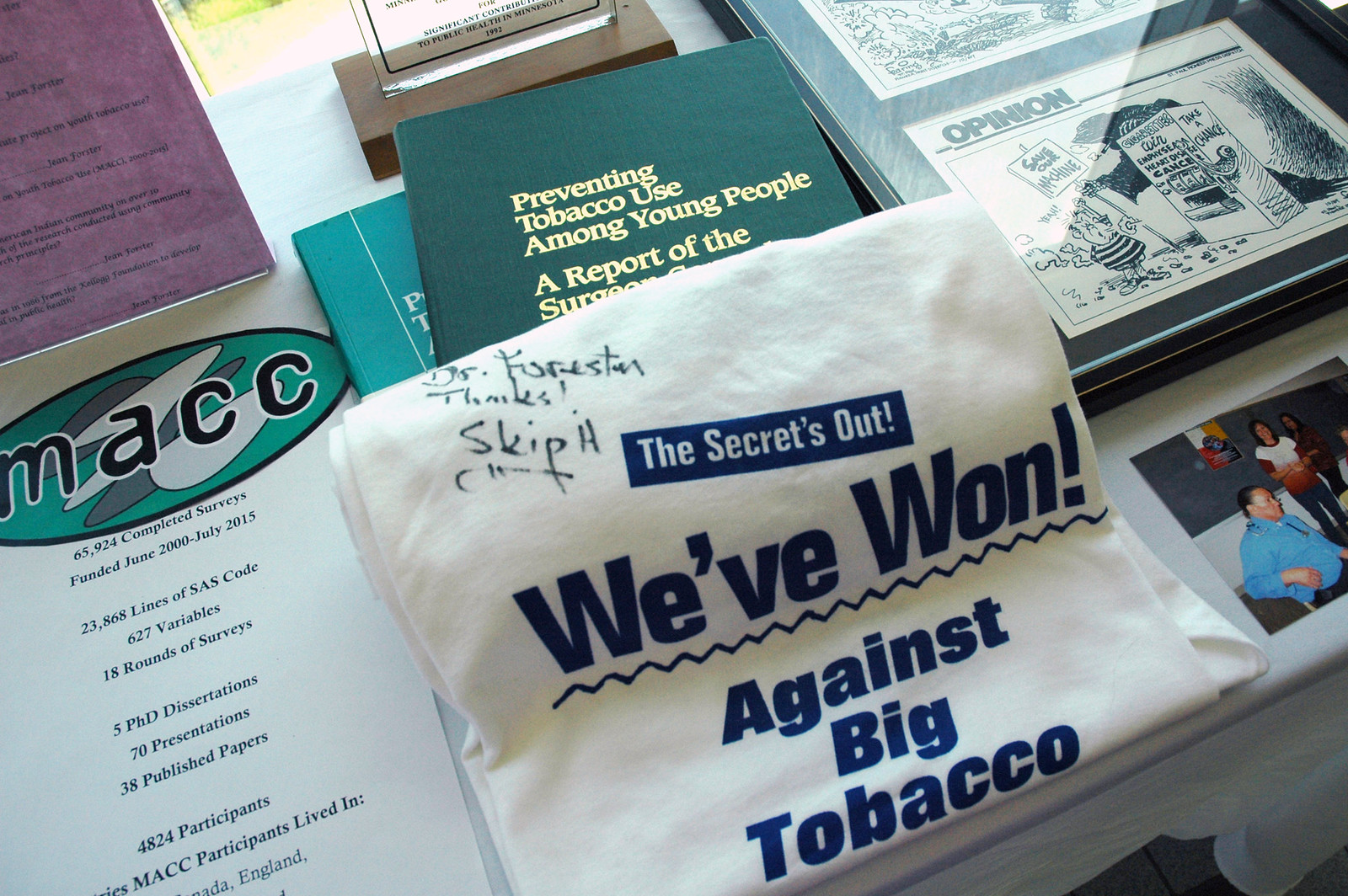The image is a detailed and eclectic tabletop spread, featuring a variety of items arranged in a somewhat disorganized manner, with everything tilted slightly upwards and to the left. On the left-hand side of the table, there is a piece of paper with the emblem "MACC" at the top, listing "Completed Surveys, Ph.D. Dissertations, Presentations, Papers." Above this paper is a purple sheet extending out of the frame.

To the right, there's a small glass trophy or award on a wooden stand. Below this, two green books are stacked, one on top of the other. The title of one book reads "Preventing Tobacco Use Among Young People, Report of the Surgeon General."

The focal point of the image is a folded shirt at the center-bottom. It's been signed with "Dr. Forrester, thanks" and features a blue box with the words "The secret's out" followed by a large proclamation "Weave one!" and curly lines, further stating "against tobacco" below.

In the upper right section of the image, a framed cartoon extends out of the frame, showing what seems to be a gambling machine with a caption "Opinions Save Our Machine." Below this, there is a Polaroid photo of three individuals, one seated with two standing behind them. The bottom right corner reveals just the edge of the table, completing the scene.